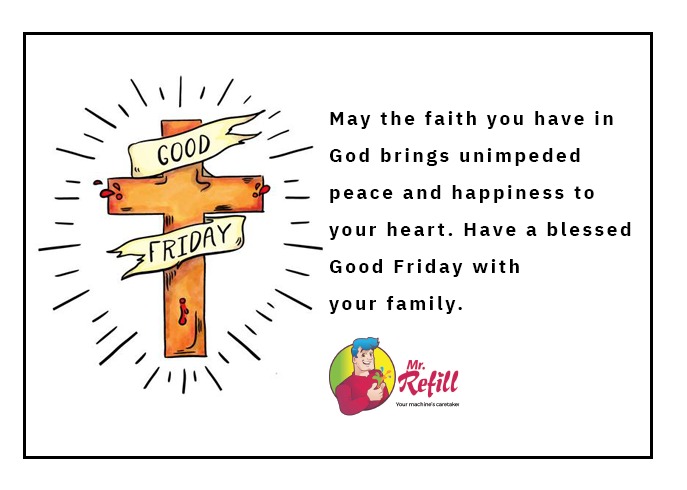The advertisement features a horizontally-aligned rectangular image bordered by a thin black line. Dominating the left side of the image is a large brown cross with streaks radiating from it, giving the impression that it is glowing. The cross has a banner split into two parts, one at the top with the word "Good" and one at the bottom with the word "Friday." Around the cross, there are dashed lines forming a circular pattern. To the right of the cross, left-aligned text in black reads: "May the faith you have in God brings unimpeded peace and happiness to your heart. Have a blessed Good Friday with your family." Beneath this text is a small circular logo depicting a smiling man with blue hair in a red long-sleeve shirt, set against a yellow and green background. The man appears to be either holding or snapping his fingers, with ink or flowers blooming from his hand. To the right of the logo, it says "Mr. Refill" in purple text, alongside a small black print reading "your machine's caretaker." The background of the entire advertisement is white.